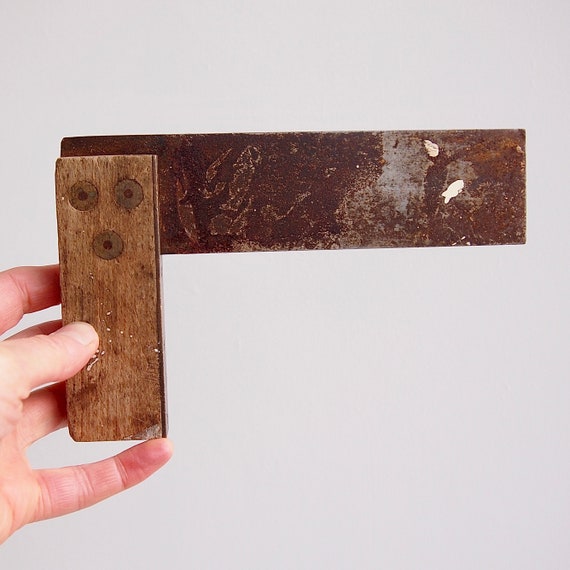In the image, a left hand, belonging to a white person, emerges from the left side, holding up an antiquated carpenter’s square. The tool's handle, crafted from lighter-colored wood, is grasped securely by the thumb, revealing three prominent gold-colored rivets. Its L-shaped metallic blade shows significant rusting, marked by a spectrum of orange and dark amber hues. Towards the left, a notable patch reveals some of the original silver-toned metal, adorned with two small white paint drops, the one at the bottom slightly brighter than the top. The badly rusted metal further features a silhouette formed by white scratch marks near the handle, intriguingly resembling a person with arms outstretched. The tool's overall ruggedness is highlighted against a soft gray backdrop, giving a stark contrast to its worn condition and the seemingly accidental white paint specks, one of which whimsically shapes a fish silhouette. The image captures the rustic essence and storied past of the square, emphasizing the detailed interplay of decay and the tool's enduring structure.